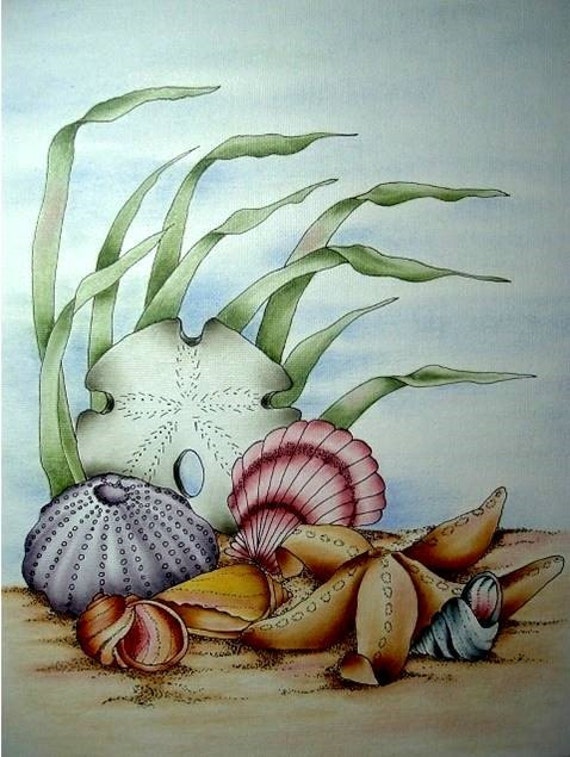This detailed illustration of underwater life features a serene scene bathed in a light blue hue, evocative of a sunlit sea. The lower third of the image is covered in a sandy terrain, where various marine elements rest. Dominating the background is a cluster of long, green seaweed blades swaying gently to the right. At the base of this underwater vegetation lies a beige sand dollar, slightly off-center to the left. 

In front of the sand dollar, there is a collection of vivid seashells and marine creatures. A light purple-gray shell sits to the far left, while a classic pink seashell, adorned with stripes and shading, is centered on the sand. Near these, a yellow seashell shape and a small, dark pink or peach sea snail shell add to the variety. 

Additionally, a starfish, illustrated in a rich orange, is lying flat, and another empty shell with a blue-gray spiral pattern is positioned at the bottom right corner. Amongst these shells, a brown seahorse and a purple sea urchin, dotted along the top, can also be seen.

This intricate artwork appears to have been created with colored pencils, giving it a textured and vibrant look. The entire scene beautifully captures the calm and diverse ecosystem of the underwater world.